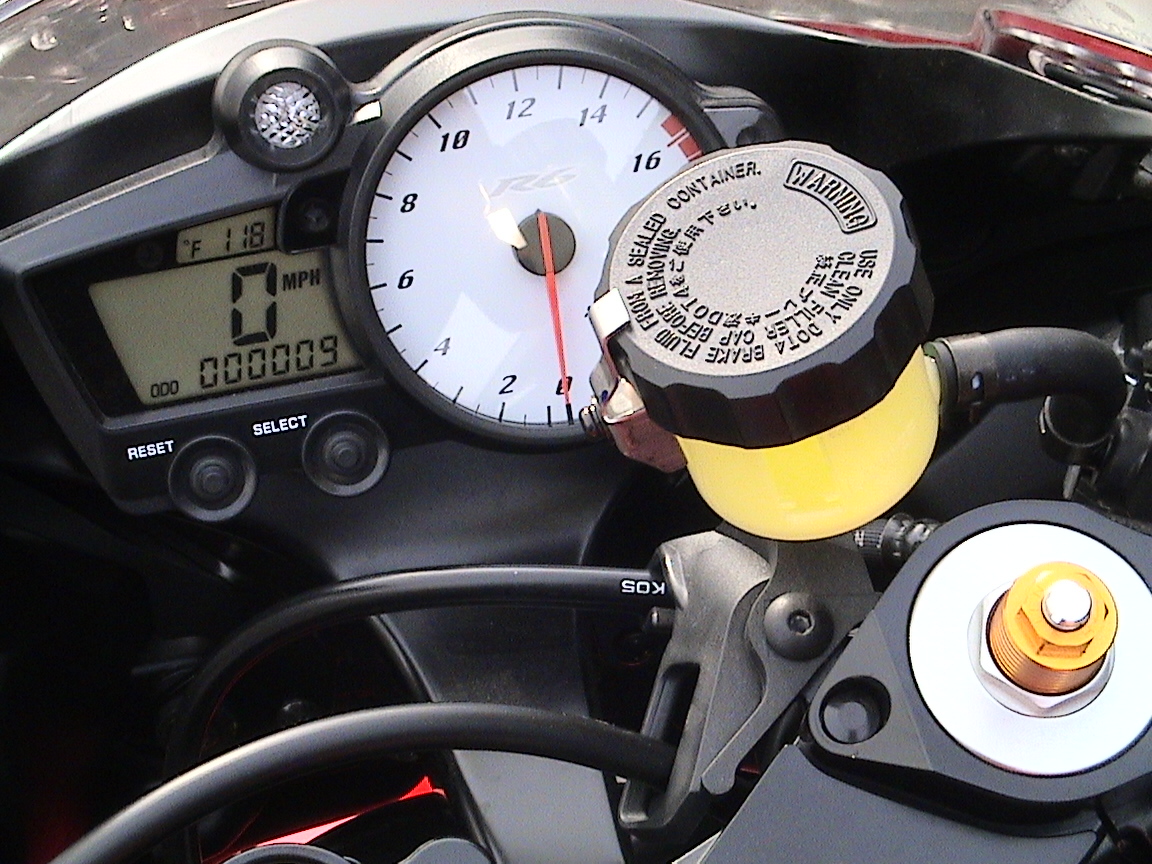The close-up image captures the intricate details of a motorcycle dashboard, predominantly black in color. At the left-center, a prominent digital display serves as the speedometer, currently reading zero miles per hour in large digits. Just below, the odometer indicates a total distance of nine miles traveled in smaller figures. Above the speedometer, a smaller rectangular display shows the temperature, a scorching 118 degrees Fahrenheit.

In the center of the dashboard resides a round RPM meter with a white face, displaying values from 0 to 16. Partially obscuring the RPM meter is a cylindrical brake fluid reservoir with a black screw cap, featuring a warning label that instructs to "use only brake fluid from a sealed container" and to "clean filter cap before removing." The same instructions are repeated in Chinese characters around the base of the reservoir. A large black hose is visibly connected to this container.

In the foreground to the left, two smaller black wires are seen connecting to a silver component. Meanwhile, in the lower right corner, there's a round silver part with a yellow, screw-like cap, characterized by a threaded appearance and a tiny silver circle on its top.

The top left and top right corners of the image reveal portions of the motorcycle's windshield, providing a glimpse of partial red detailing that hints at the motorcycle's overall color.